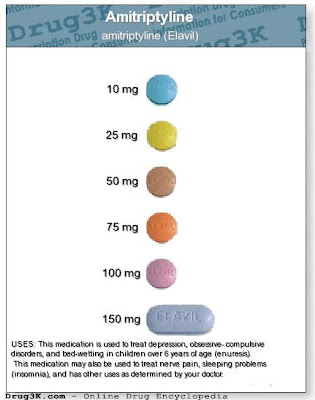The top section of the image features a teal-colored banner with the text "DRUG3K" followed by the words "for consumers." 

In the central white section, the primary focus is on the medication named "Amitriptyline," with the brand name "Elavil" written in parentheses below it. The text specifies varying dosage forms of the medication, displayed within colored circles: 
- A blue circle labeled "10 mg"
- A green circle labeled "25 mg"
- A brown circle labeled "50 mg"
- An orange circle labeled "75 mg"
- A purple circle labeled "100 mg"
- A light purple oval labeled "150 mg"

This section also provides information about the uses of Amitriptyline (Elavil), stating that the medication is prescribed for treating depression, obsessive-compulsive disorders, and bedwetting in children over six years old. Additionally, it mentions that the medication may be utilized to address nerve pain, sleeping problems (insomnia), and other conditions as determined by a doctor.

At the bottom, the image references the source "drug3k.com - online drug encyclopedia."